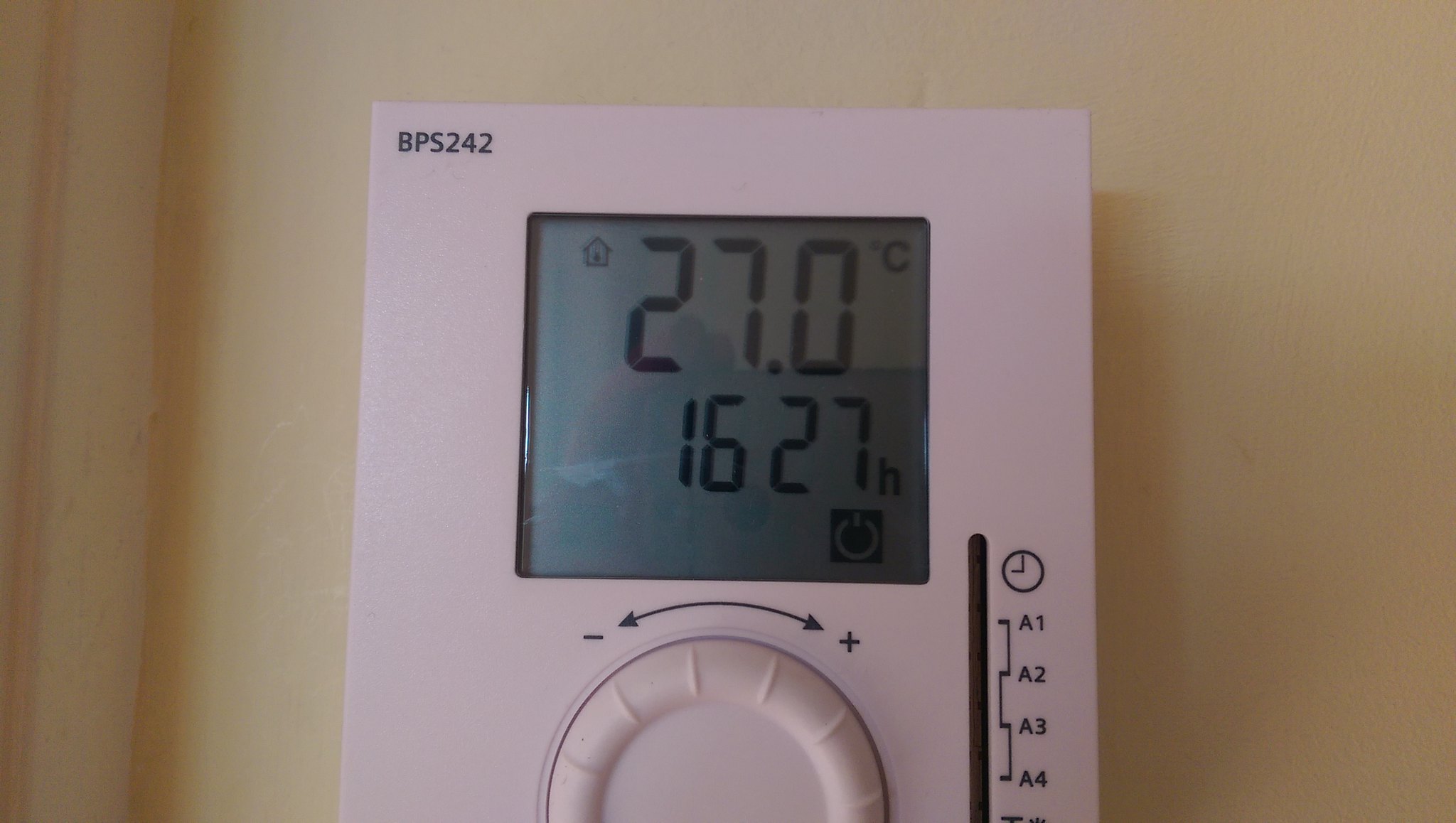This photograph features a white, rectangular thermostat, designed for regions that utilize Celsius for temperature measurement and military time for the clock display. Prominently displayed in the top left corner of the thermostat are the prominent letters "BPS" and the number "242." The thermostat includes a white, rotatable knob at the bottom, which can be turned to the left for decreasing values (indicated by a negative sign) and to the right for increasing values (indicated by a positive sign). Above this knob, these directional instructions are clearly printed for user convenience.

To the right of the knob, there is a vertical line featuring a clock icon, followed by labels "A1," "A2," "A3," and "A4" directly beneath it. Central to the device is a digital display screen, which currently shows the temperature as 27.0 degrees Celsius and the time as 16:27 hours. In the bottom right corner of this display, a power icon is visible, suggesting the presence of a power mode. Additionally, a small house icon appears in the top left corner of the screen, possibly indicating that the device is in "home" or "default" mode.

Overall, the image captures a detailed view of a thermostat, clearly indicating both the current temperature and time, and illustrating the interface for user operation.